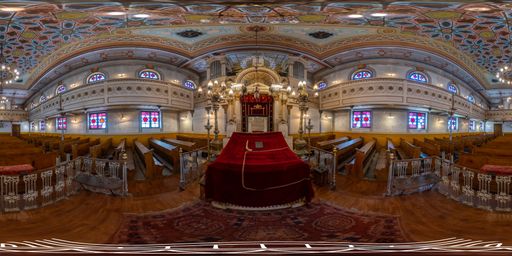The image depicts the interior of a church or cathedral, showcased in a panoramic view. Dominating the center is a structure enveloped in dark red velvet fabric, which might be a table or platform. Surrounding this centerpiece are rows of church pews crafted with intricate metalwork, possibly fencing around the central object or as part of the benches. The walls are adorned with numerous stained glass windows, approximately eight on each side, in hues of pink, blue, purple, and red. The ceiling is richly decorated, featuring a kaleidoscope of floral patterns and detailed designs in blues, purples, and golds. The scene is illuminated by lights that accentuate the stained glass and the ornate ceiling. The floor, appearing wooden, is partially covered by what seems to be an oriental rug in front of the red-velvet-clad structure. White walls and additional gold trim add to the opulent atmosphere of the space.